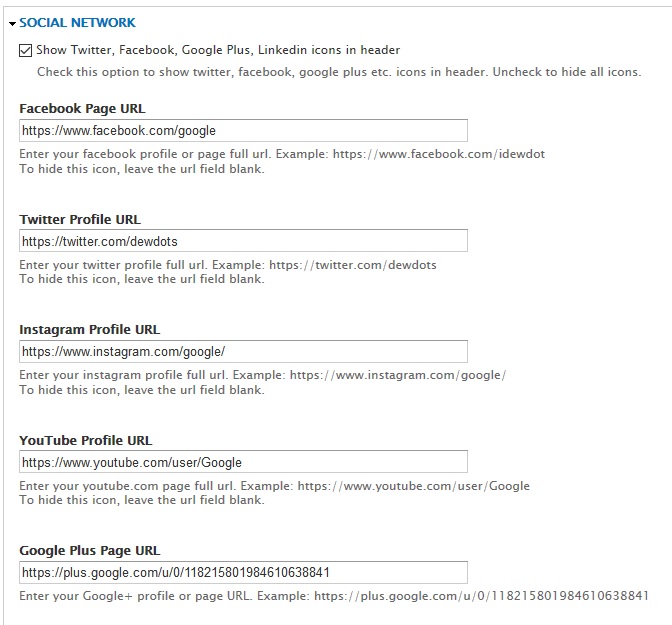The image depicts a screenshot from a website interface displaying various settings for social media integration. At the top, there is a thin line running across the screen horizontally, and another thin line descends vertically along the left side. Prominently, at the top of the interface in bold blue capital letters, the text "SOCIAL NETWORK" is displayed, accompanied by a small black arrow pointing downward.

Beneath the "SOCIAL NETWORK" heading, there is a checkbox with a thin black checkmark inside it. Next to the checkbox, the text reads: "Show Twitter, Facebook, Google+, LinkedIn icons in header. Check this option to show Twitter, Facebook, Google+, etc., icons in the header. Uncheck to hide all icons."

Following this section, there are fields for entering URLs of different social media profiles, each accompanied by instructional text and example URLs. The first field, labeled "Facebook Page URL" in dark text, is intended for users to enter the full URL of their Facebook profile or page. It includes an example URL and notes that leaving this field blank will hide the Facebook icon.

Next is the "Twitter Profile URL" field, which similarly prompts users to enter their complete Twitter profile URL, providing an example and instructions to leave the field blank to hide the icon.

The subsequent field is for the "Instagram Profile URL." This field is pre-populated with a placeholder web address and includes the same type of information: a prompt to enter the full URL of the Instagram profile, an example, and a note about hiding the icon if left blank.

Following that is the "YouTube Profile URL" field, also pre-populated with a placeholder URL. Users are instructed to enter their full YouTube page URL and are reminded that they can hide the icon by leaving the field blank.

Lastly, the "Google Plus Page URL" field, similarly populated, asks for the full URL of the user's Google Plus profile or page, complete with an example and the option to hide the icon by not entering a URL.

Each profile section maintains a consistent format of entry prompt, example URL, and instructions for hiding the respective icons if the fields are left blank. This detailed interface allows users to configure the visibility and links to their social media profiles directly within the website's header.